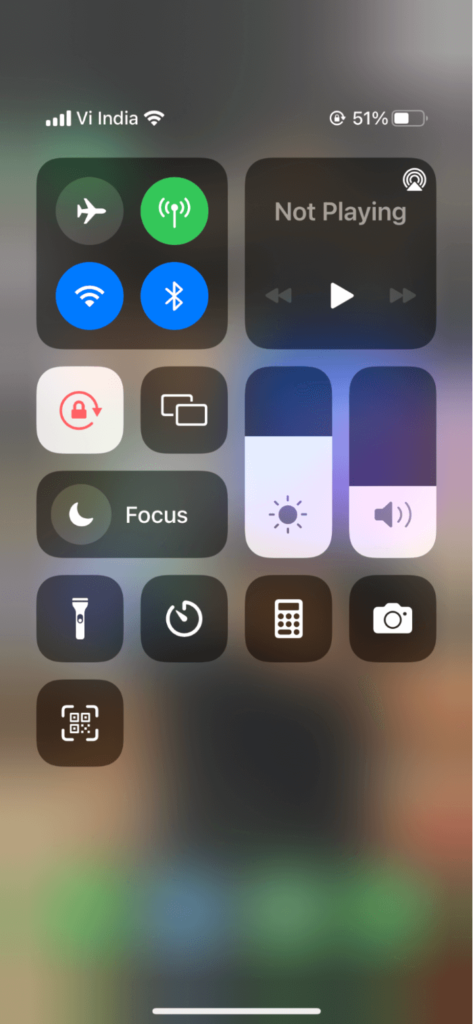The image depicts a screenshot of a smartphone interface, focusing on various control settings and notifications. At the top left corner, the status bar shows the "VI India" network along with the battery level at 51% and active Wi-Fi connection. Directly below the network status is a grid of four control icons. The first icon in the grid displays an airplane symbol indicating Airplane Mode, the second represents Wi-Fi, the third is for Bluetooth, and the fourth icon, encased in a green circle, appears to be for mobile data.

To the right of these icons, there is a "Now Playing" box featuring a play button, with navigation arrows for both backward and forward actions. Underneath this section is another set of controls starting with a white box that has a red lock icon accompanied by a refresh symbol to its right. Next to this is a black square containing two white boxes below it, indicating the Focus Mode button. 

Further down, there is a series of quick access tools: a flashlight icon, a QR code reader, a clock for setting time, a calculator, and a camera icon. Directly beneath these icons, the display shows a brightness slider which is slightly over half-full, indicated by a white bar. Adjacent to it, a volume bar is set to approximately 40%. Additionally, the battery life is again displayed in white, reinforcing its visibility.

In the background of the interface, there are various blurred floating app boxes and icons, mostly in green except for the second one from the left, which is blue. These icons are not legible due to the blur, making it difficult to discern the specific applications they represent.